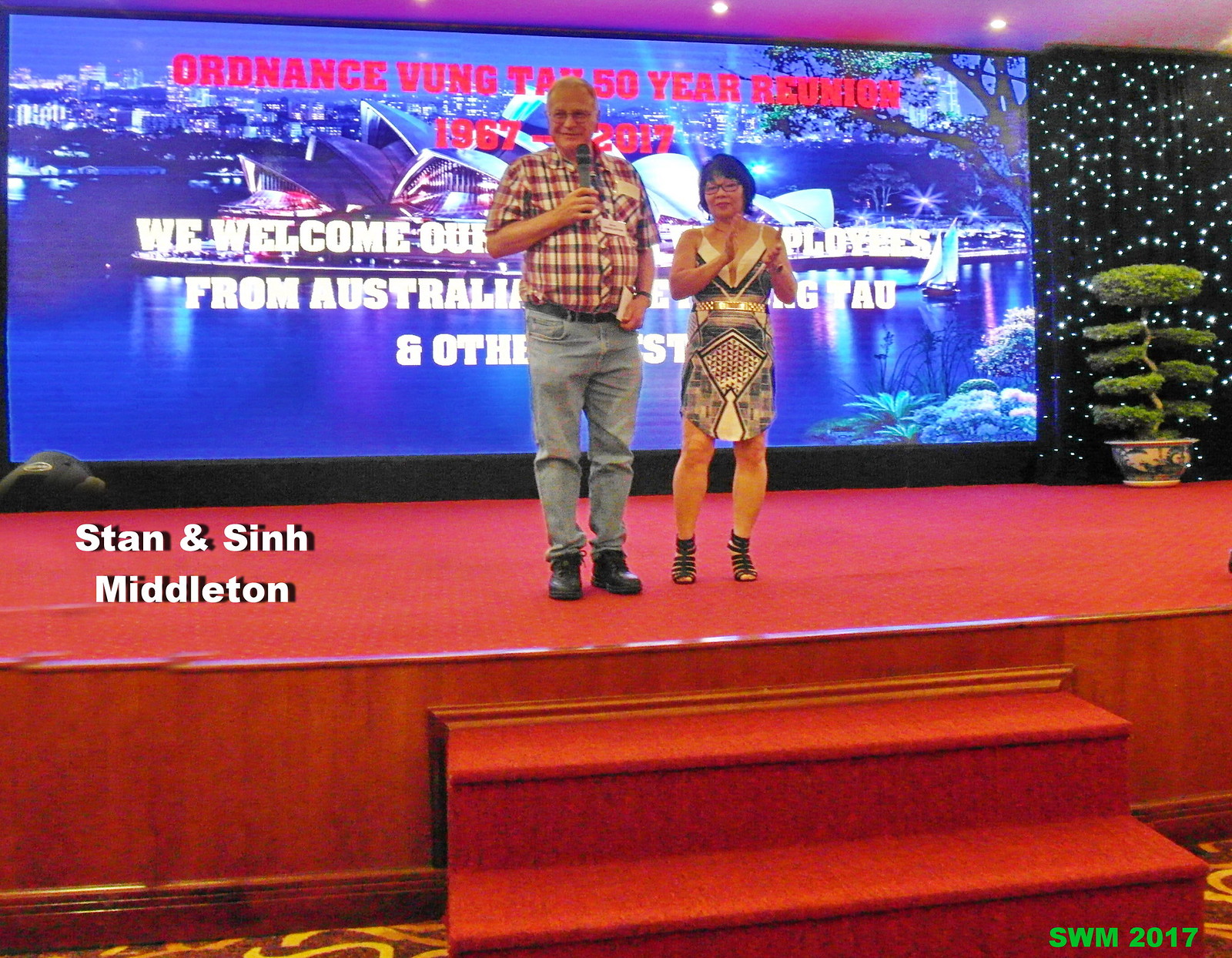This image captures a moment on stage featuring a European man and an oriental woman at the Ordinance Fung Tau 50-Year Reunion, held from 1967 to 2017. The stage, adorned with a red carpet and two sets of stairs, sets a regal atmosphere. Behind the duo, a large screen displays the event's name in striking red letters, partially obstructed by the individuals standing in front of it. A white font to the left of the screen reads, "Stand and Sing Middleton." To the right, a bonsai-like tree decorates the scene, juxtaposed against a black backdrop studded with various white lights.

The man, equipped with a microphone and some note cards in his left hand, wears a casually stylish ensemble of blue jeans, a plaid short-sleeve shirt in red, white, and blue, a belt, and boots. The woman, beside him, sports an eye-catching sleeveless dress with funky, superhero-esque designs, complemented by glasses and strappy black sandals.

Both seem engaged with the audience, the man mid-speech, and the woman clapping energetically. The scene exudes a sense of celebration, history, and community as they stand united on the festively adorned stage.